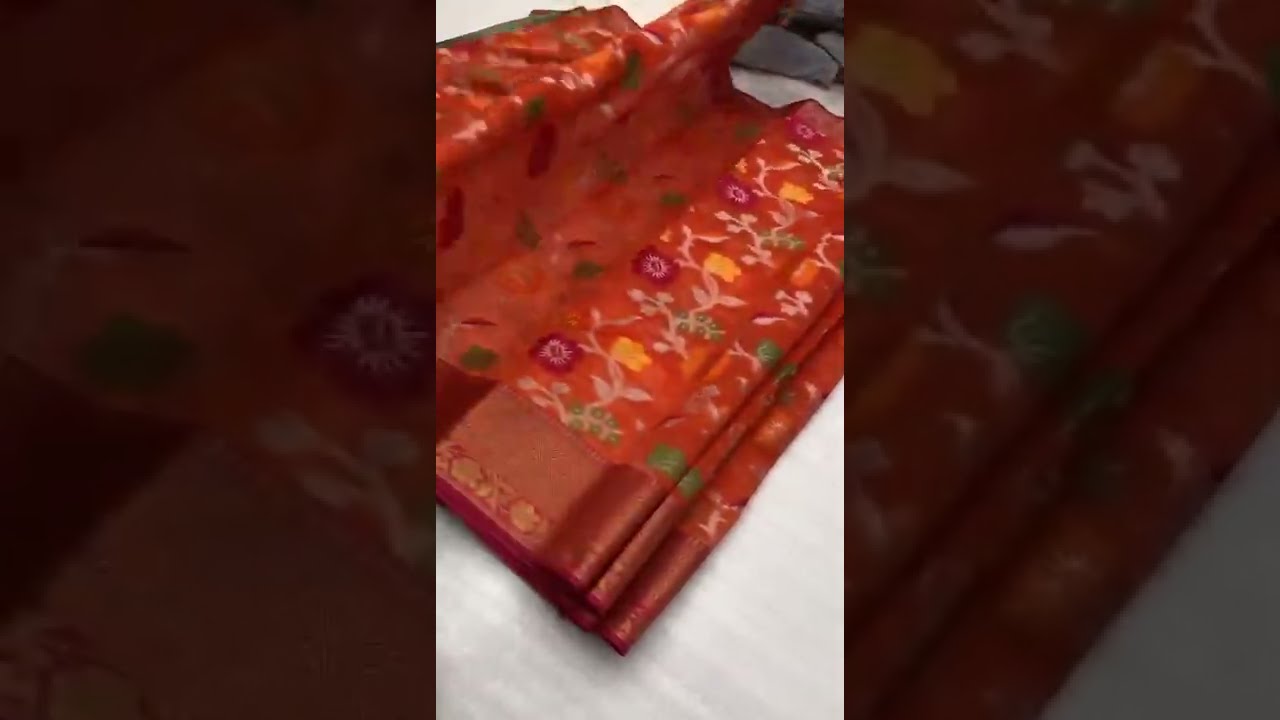The image features a wide rectangular composition centered around a tall vertical photograph of a piece of fabric, which is slightly scrunched up at the sides and extends from the bottom middle to the top left and right corners. The fabric is red with a detailed pattern of beige vines interwoven with yellow, green, and maroon flowers. This central photograph sits on a light gray surface that resembles synthetic wood. Flanking the main photo are cropped, much darker, close-up sections of the same fabric, giving a zoomed-in view of the floral pattern. The fabric appears to be either part of a curtain or an Asian-style garment, folded and resting on the ground. Additional bolts of fabric, stacked and partially unrolled, are visible, suggesting multiple layers and pieces in the frame. Overall, the design and layering of the image, combined with the floral motifs and red fabric, offer a rich visual depth and intricate detail.